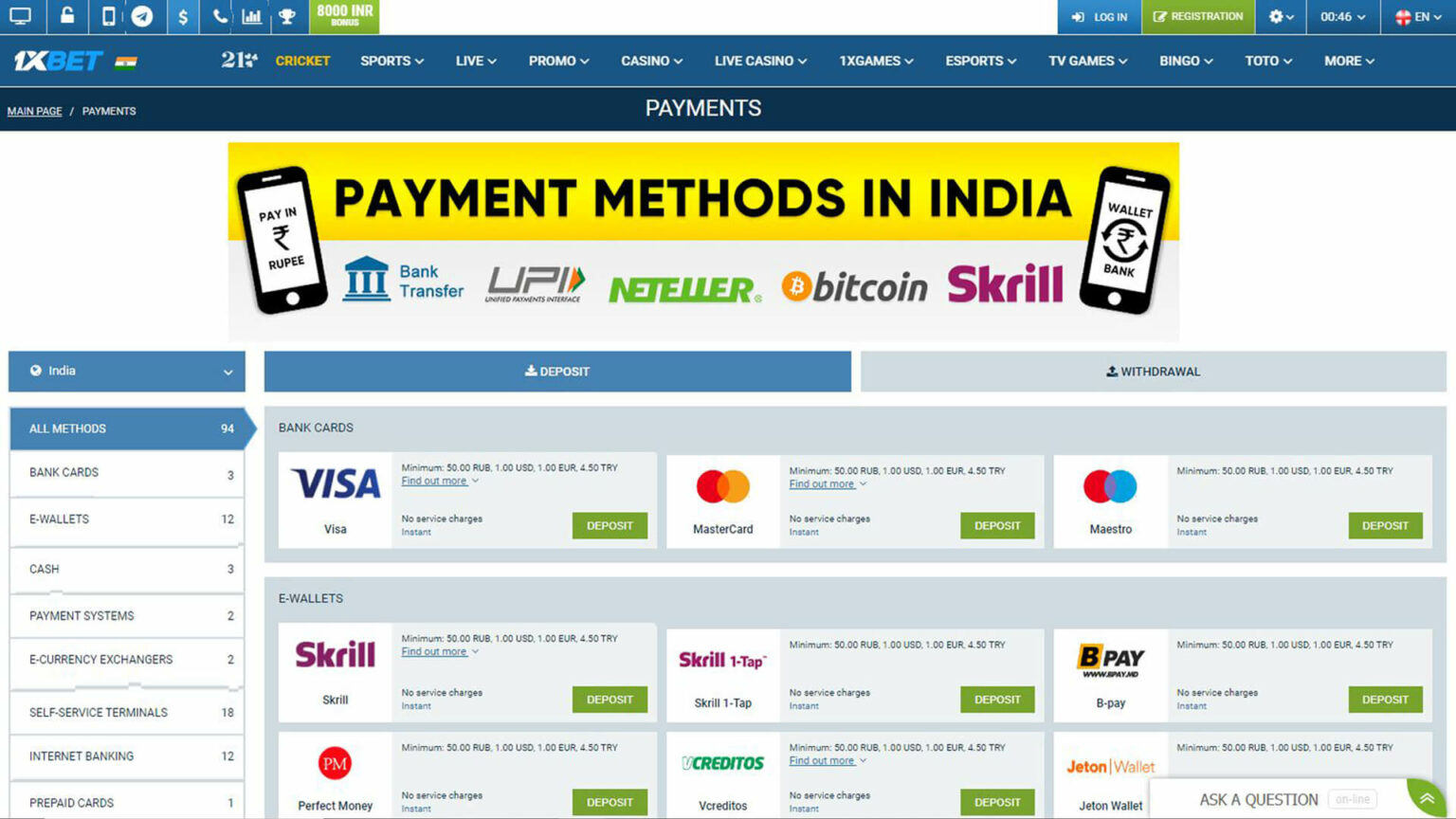This is a detailed screenshot from the 1xBet website, which appears to be a platform offering various financial services, resembling a mobile banking application. Prominently displayed under the main header is a vibrant yellow banner, which effectively grabs attention with its bold black text stating "Payment Methods in India." The banner highlights multiple payment options available to users, including Bank Transfer, UPI, Neteller, Bitcoin, and Skrill.

On the left side of the screen, there is a comprehensive menu listing all the financial services supported by the website. These include bank cards, e-wallets, cash transactions, payment systems, e-currency exchanges, self-service terminals, internet banking, and prepaid cards, providing users with a plethora of options to choose from.

The right-side pane is designed for quick access to essential features, featuring prominent "Deposit" and "Withdraw" buttons for user convenience. This section also showcases various types of bank cards and e-wallets, ensuring users have immediate access to the most relevant financial tools.

Overall, the layout is user-friendly, with a clear focus on providing a wide range of payment methods, catering specifically to the Indian market.